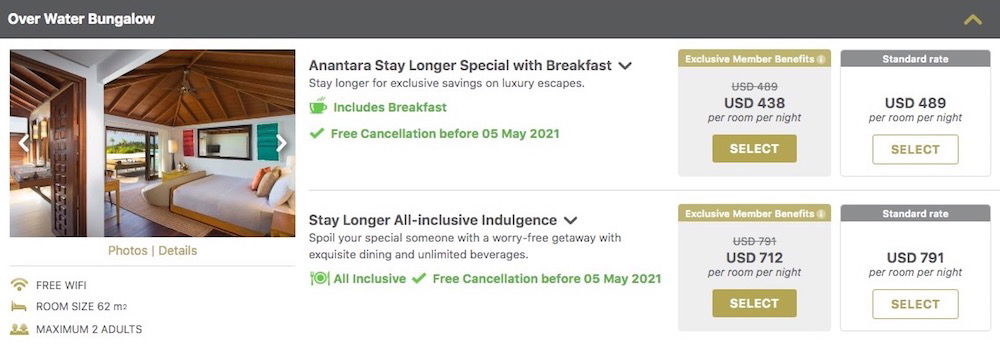This image showcases a meticulously cropped screenshot of a web page featuring luxurious holiday accommodations. The webpage's opulent design employs a refined color palette of greys, whites, and golds, exuding a sophisticated ambiance. Dominating the top of the image is a dark grey rectangular box with the header “Overwater Bungalow.” 

Beneath this header, detailed information about the Overwater Bungalow is presented, accompanied by an enticing image depicting the chic interior of the bungalow at a plush poolside summer resort. Two deluxe accommodation options are highlighted: 

1. **Antara Stay Longer Special with Breakfast**:
   - **Member Rate**: $438 per night
   - **Standard Rate**: $489 per night

2. **Stay Longer All-Inclusive Indulgence**:
   - **Member Rate**: $712 per night
   - **Standard Rate**: $791 per night

Both options suggest an exceptional level of luxury, with the first being inclusive of breakfast, while the second offers an all-inclusive dining experience, catering to guests seeking a supreme vacation experience.